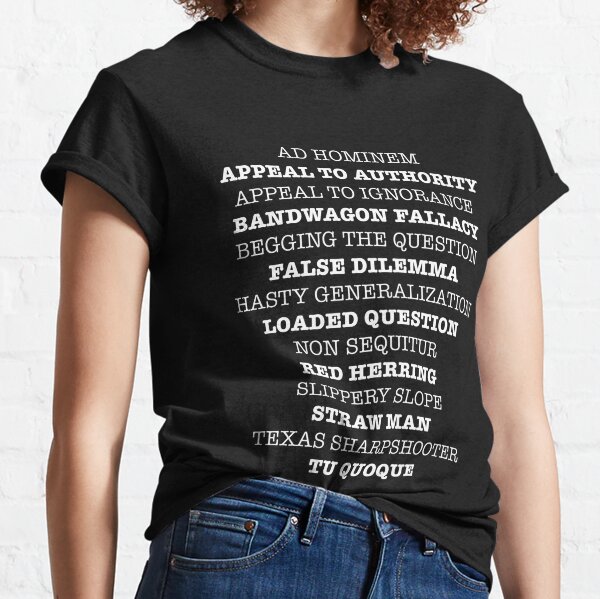This color photograph features the torso of a Caucasian woman standing leisurely, with dark, shoulder-length curly hair, wearing blue jeans, and a black t-shirt with short sleeves rolled up. The t-shirt is the focal point of the image and is adorned with a detailed white text print listing various logical fallacies: "ad hominem, appeal to authority, appeal to ignorance, bandwagon fallacy, begging the question, false dilemma, hasty generalization, loaded question, non sequitur, red herring, slippery slope, straw man, Texas sharpshooter, and tu quoque." The image is composed to highlight the t-shirt, making it appear as if it could be an advertisement for it.